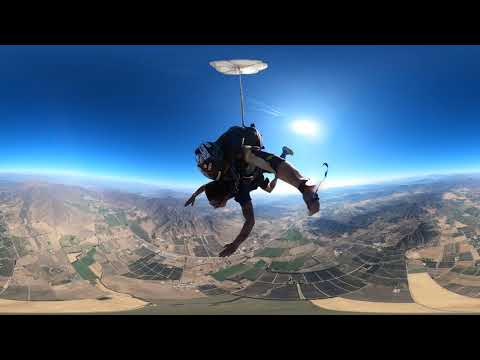The image captures an exhilarating skydiving moment framed with thick black borders at both the top and bottom. At the center of the image, high in the air against a deep blue sky, two people are in the midst of their dive. The primary focus is on the duo, where one person is positioned on the back of the other. The person on the bottom, light-skinned with arms fully extended forward in a Superman-like pose, faces slightly towards the viewer and to the left, displaying a body adorned with tattoos. The person on top is facing left, with their legs hanging down and equipped with a parachute strapped to their back, featuring an unusual extension with a white, circular end that may be the beginning of the parachute deployment. Below them, an expansive and vividly detailed landscape shows a hilly and mountainous terrain divided into rectangular parcels of green and brown fields, evoking the impression of soaring high above the earth. The scene is bathed in daylight, with a bright, spherical sun visible in the background, providing a clear, breathtaking view of the skydiver's daring plunge.